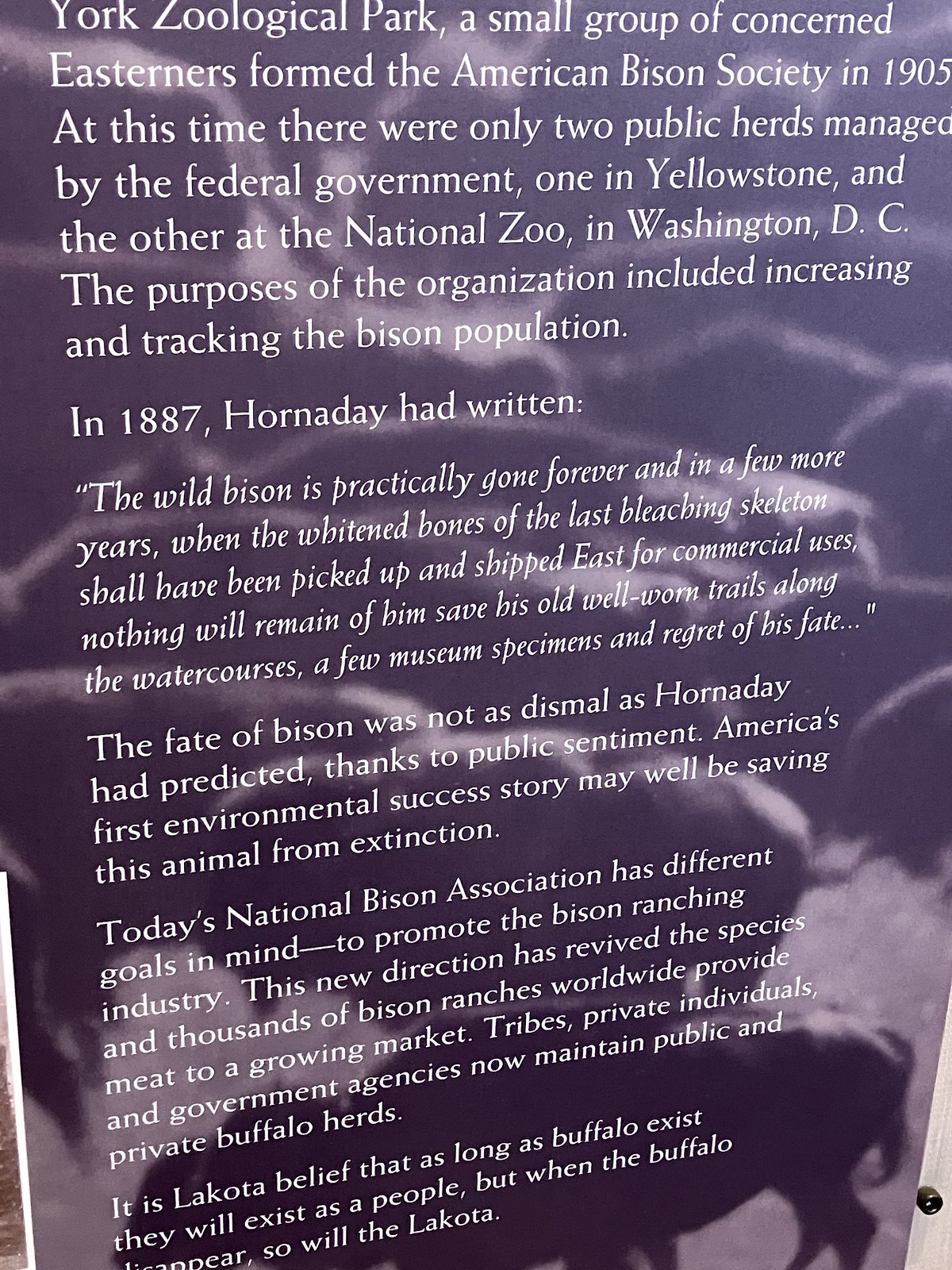The image showcases a poster with a blurred, purple-toned background featuring animals with four legs and tails, likely bisons. The poster appears to be a museum or zoo placard, given the detailed historical content it bears. The text, left-justified in white and spread across six paragraphs, discusses the formation and efforts of the American Bison Society, founded by concerned Easterners in 1905. At that time, only two public bison herds existed, in Yellowstone and the National Zoo in Washington, D.C. The purpose of the society was to increase and track the bison population. One paragraph includes a quote from Horan Day in 1887, lamenting the near extinction of wild bison but noting the subsequent conservation success. The text also references a belief attributed to Lakerton about the intertwined fate of the bison and the Lakota people. A notable detail is that one paragraph is in double quotations and written in a different font. The poster, likely located on a white door (evidenced by a visible doorknob in the lower right), is a testament to America's early environmental efforts to save the bison from extinction.